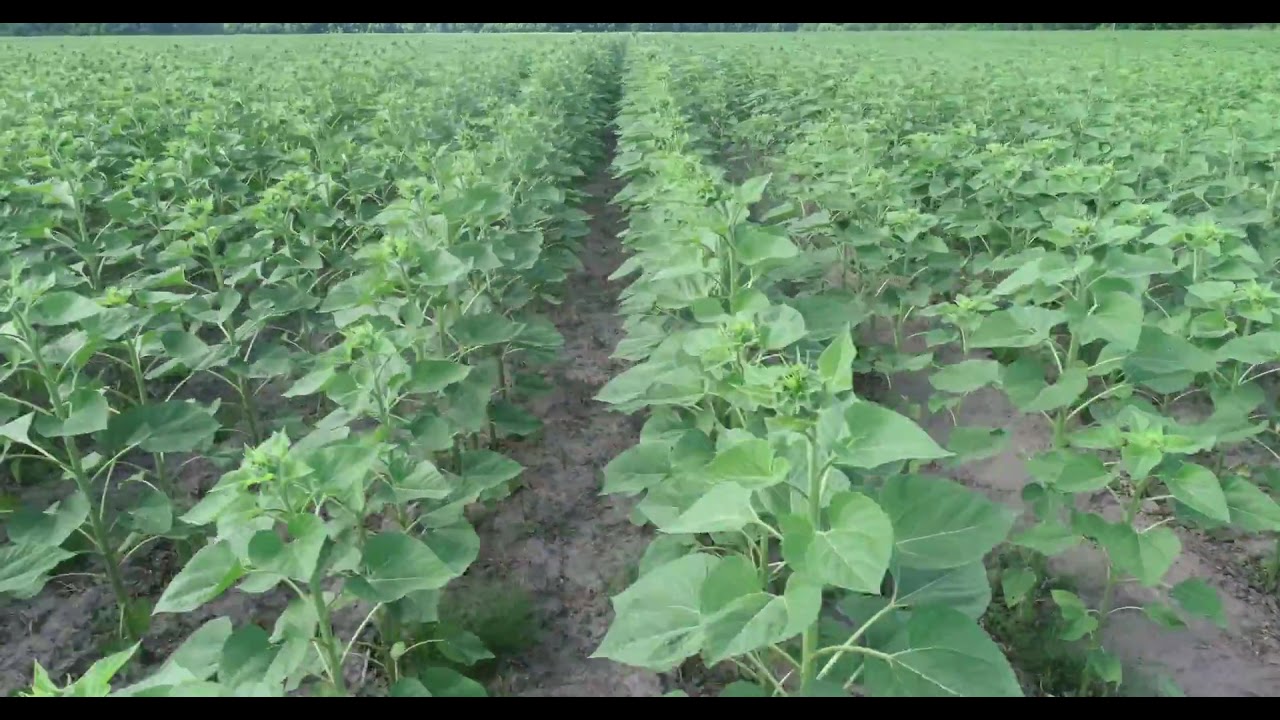This is a rectangular photograph of a vast crop field, characterized by an array of uniform green plants standing approximately 15 inches tall. These plants, adorned with large, bright green leaves, are systematically arranged in rows stretching from the foreground to the horizon. Each row is separated by visible gray dirt, highlighting the orderly structure of this farm. At the tops of the plants, there are distinctive blooms resembling balls comprised of various shades of green, with delicate hair-like growths emerging from each bulb. The bottom right corner of the image shows a few weeds encroaching near some of the rows. The photograph is framed by two horizontal black bands at the top and bottom, creating a striking contrast against the abundant greenery within the field. In the distance, a thin line of additional brush can be seen, marking the farm's boundary.